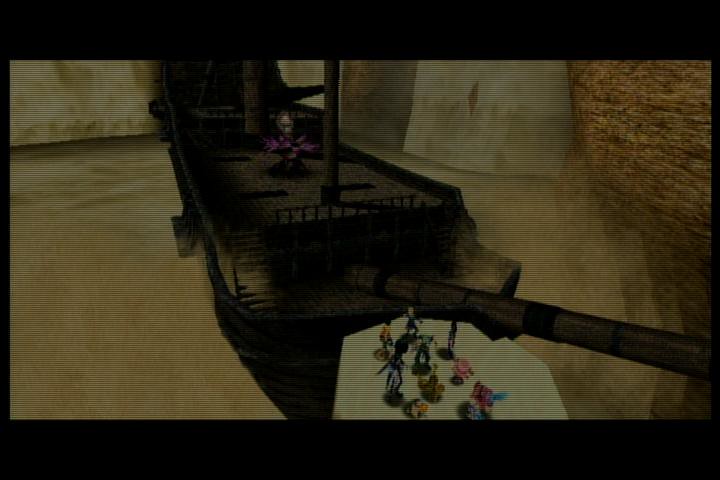This is a colored photograph of a video game screen showing a large pirate-esque ship viewed from a slightly three-quarter angle of the bow and deck. The ship, shaded in charcoal black and grey, features a prominent bowsprit extending diagonally out the lower right corner. The deck is occupied by two masts extending vertically out of the frame. The ship's stern is engulfed in darkness, providing no discernable details. Surrounding the vessel are rock walls resembling a wooden stone cliff or cave, with darkish brown hues adding to the dimly lit ambiance. In the foreground, on the forepeak, lies an octagonal white platform populated by a diverse collection of digital characters—approximately nine in total. These figures vary in size, height, and color; notable ones include a pink character, a tall and skinny black figure, an even taller blue character with white pants wielding a sword, a small orange and yellow character, and another vibrant mix of red, blue, and yellow. The image lacks any text or print, focusing solely on the detailed digital scene.